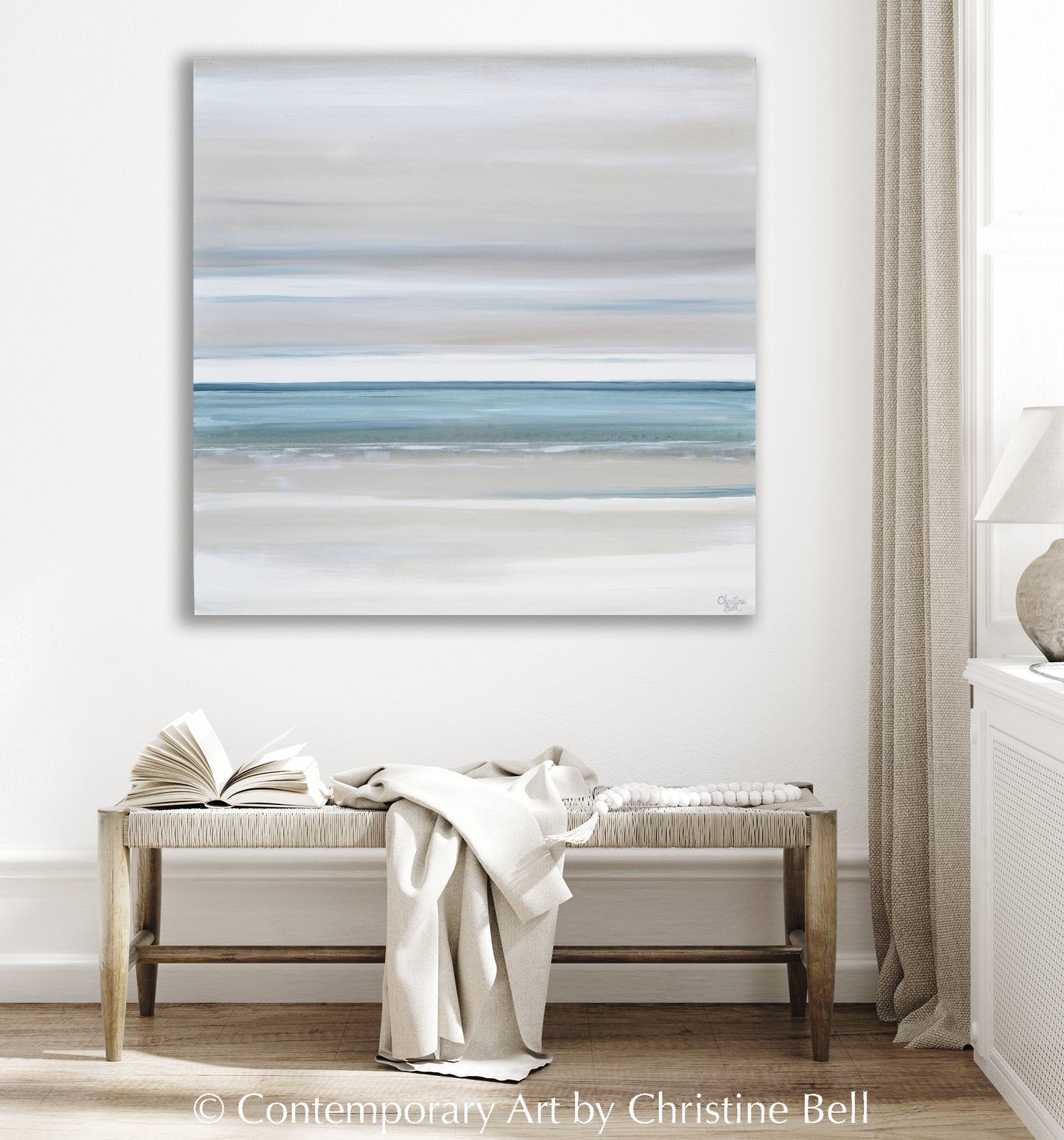In this interior scene resembling a styled product display, a large, square painting titled "Contemporary Art by Christine Bell" anchors the composition, mounted on a pristine white wall. The painting, which depicts a beach and ocean, shows the shore transitioning from white to tan as it meets small, gentle waves. Tan and dark grey clouds with hints of blue scatter across the cloudy sky. A small round lamp with a white lampshade sits to the left of the painting, while tan window shades and a curtain frame a window to the right, reinforcing the coastal theme. Below the painting, a rattan bench adorned with a neatly folded blanket, an open book, and an artistic bead arrangement completes the serene setup. A watermark featuring a 'C' in a circle and "Contemporary Art by Christine Bell" is subtly placed at the bottom of the painting, adding a professional touch.